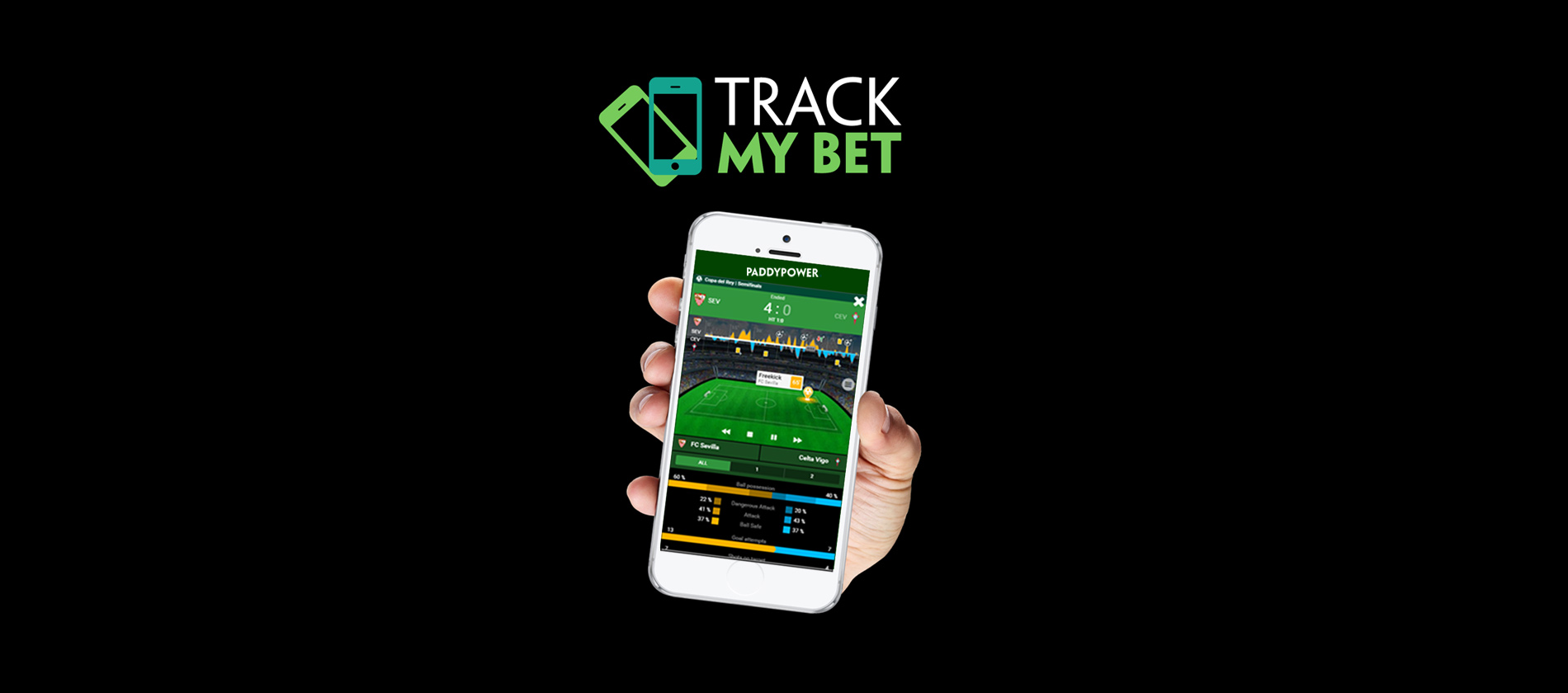This advertisement for a sportsbook app is displayed on a long horizontal rectangle with a pure black background. Prominently in the center is a light-skinned hand holding a white mobile phone. The screen of the phone shows an image of a field, likely a soccer or football stadium, along with some unreadable statistics in blue and orange at the bottom. Above the phone, the text "TRACK" in white and "MY BET" in light green are displayed. To the left of this text is the app's logo, featuring two overlapping cellphone icons, one in light green and the other in aqua-green. The overall color scheme includes black, white, green, blue, orange, and gray, emphasizing a modern and sleek design perfect for mobile sports tracking.